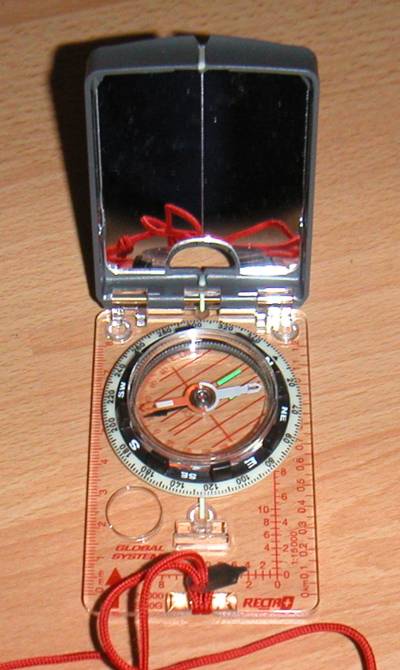The image showcases a rectangular, plastic compass device placed on a light brown table. The compass has an open black lid, which features a mirror on its underside. In the reflection of the mirror, a red string is visible near the bottom edge of the frame. The main body of the compass consists of clear plastic, with a red ruler running along the right edge and the bottom edge.

At the base of the compass, a red string is tied and extends outward. The central portion features a circular compass. Encircling the compass is a black band marked with cardinal and intercardinal directions: North (N), South (S), East (E), West (W), Southwest (SW), Northeast (NE), Northwest (NW), and Southeast (SE). Inside this black band, a white band is marked with numerical degrees.

The compass needle comprises two hands: a red-and-white hand and a green hand, both indicating the direction.